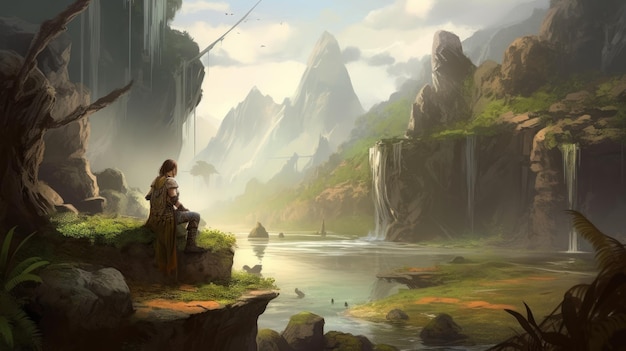This is a highly detailed digital artwork resembling a video game landscape. The scene features a tranquil body of water, likely a small pond or river, situated at the center. Waterfalls cascade from elevated rocky terrain into the water, creating ripples upon the surface. The landscape is lush with greenery, covering the hillsides and rocky outcrops with various shades of browns, grays, and greens.

In the far distance, two sharp, misty mountain peaks rise dramatically into a blue sky adorned with white clouds. Among the greenery stands a solitary tree. To the left of the image, an individual clad in warrior-like attire is positioned on a raised rock, one leg propped up as they gaze contemplatively over the water. The detailed illustration captures the serene yet majestic essence of the natural landscape, providing an immersive visual experience.